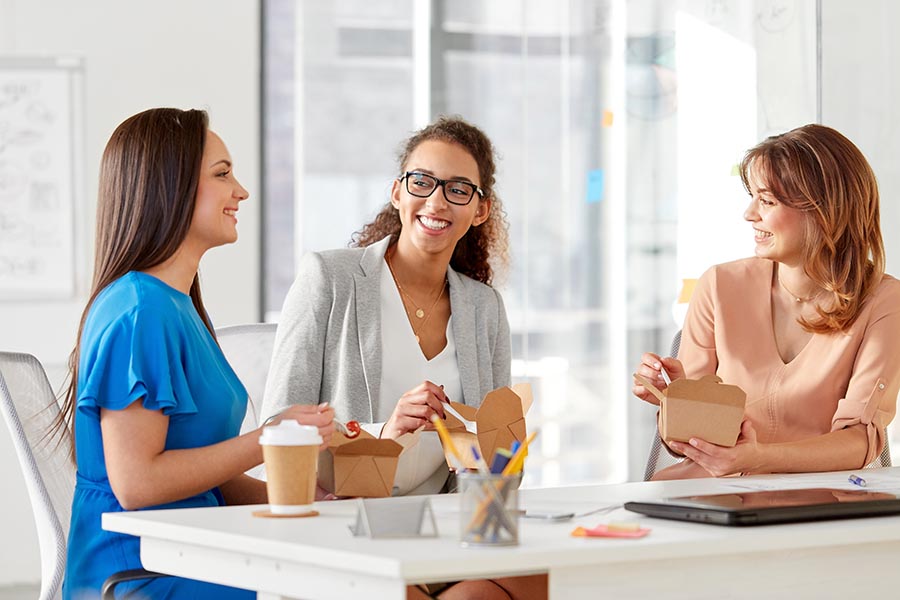Three professionally dressed young women are sitting at a polished, quartz-surfaced table, casually eating lunch and engaging in conversation. The woman on the left, with long brown hair, is wearing a vibrant blue dress and looking towards her right. The middle woman, a light-skinned Black woman with curly hair, wears a gray blazer over a white dress and sports black-rimmed glasses. She is smiling warmly. The woman on the right has dirty blonde hair and is dressed in a peach-colored blouse; she exudes a motherly vibe and is looking to her left, also smiling. They are each holding a fork and eating from brown box containers that likely contain salad and Chinese food. In addition to their meals, the table features a white desk in the foreground, a metal pencil holder with various pens and pencils, a small name tag holder or business card holder to the left, and an iPad to the right. The setting—a brightly lit office space with large windows that let in plenty of natural light—suggests they are on a break.